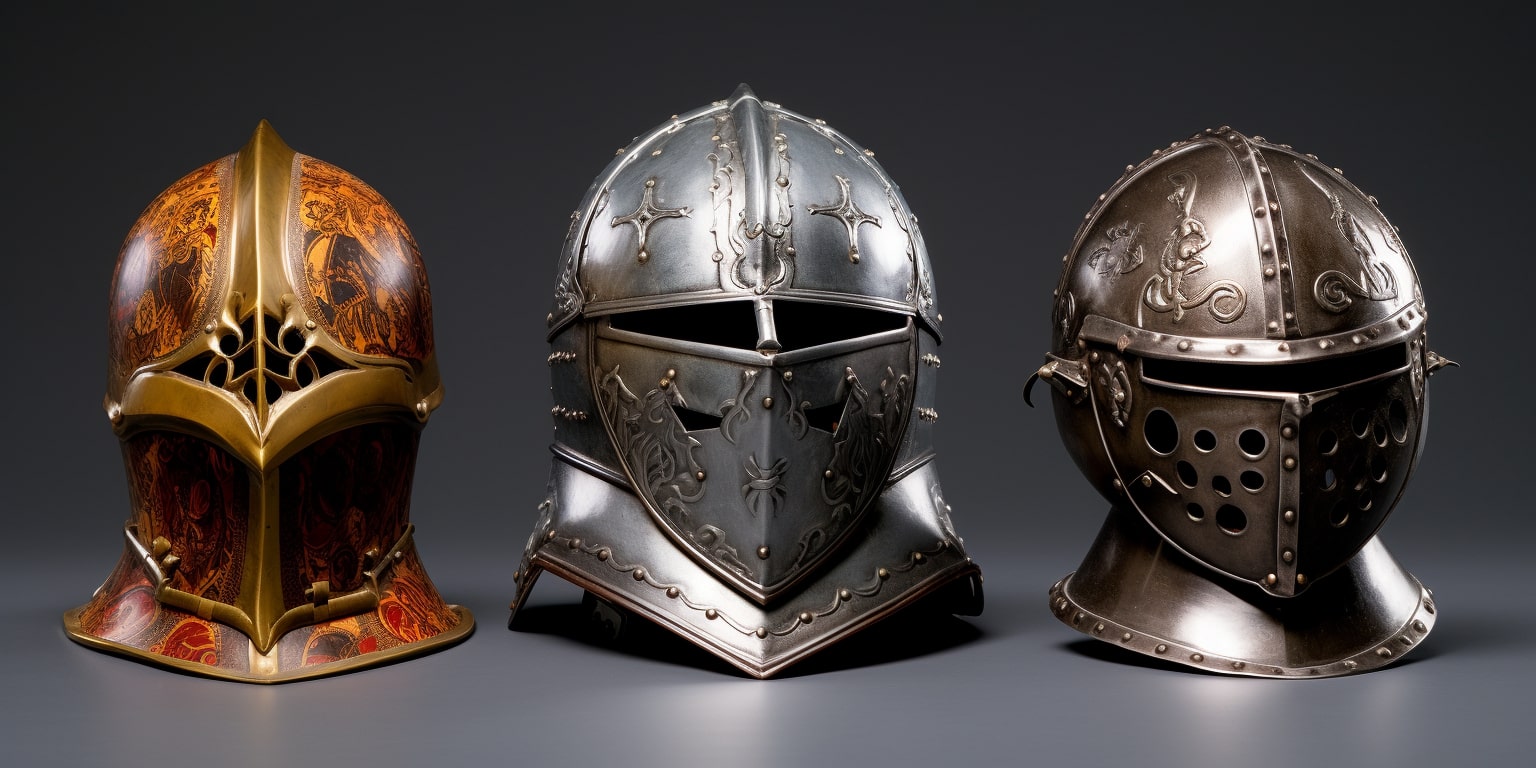This image showcases three intricately designed knight helmets set against a black background. On the left, there is a golden helmet with an open face design adorned with an elaborate mix of orange, black, gray, brown, and red paint, featuring decorative imagery along the sides. The center helmet is a sleek silver-gray steel piece, with slits where the eyes should be and small ventilation holes, exhibiting a simple yet elegant metallic finish. The rightmost helmet, a pewter or dark brown hue, is distinguished by numerous holes on the faceplate, particularly around the cheeks, contributing to its unique aesthetic. All three helmets are full-face coverings made of metal, each showcasing a distinctive style and color pattern.